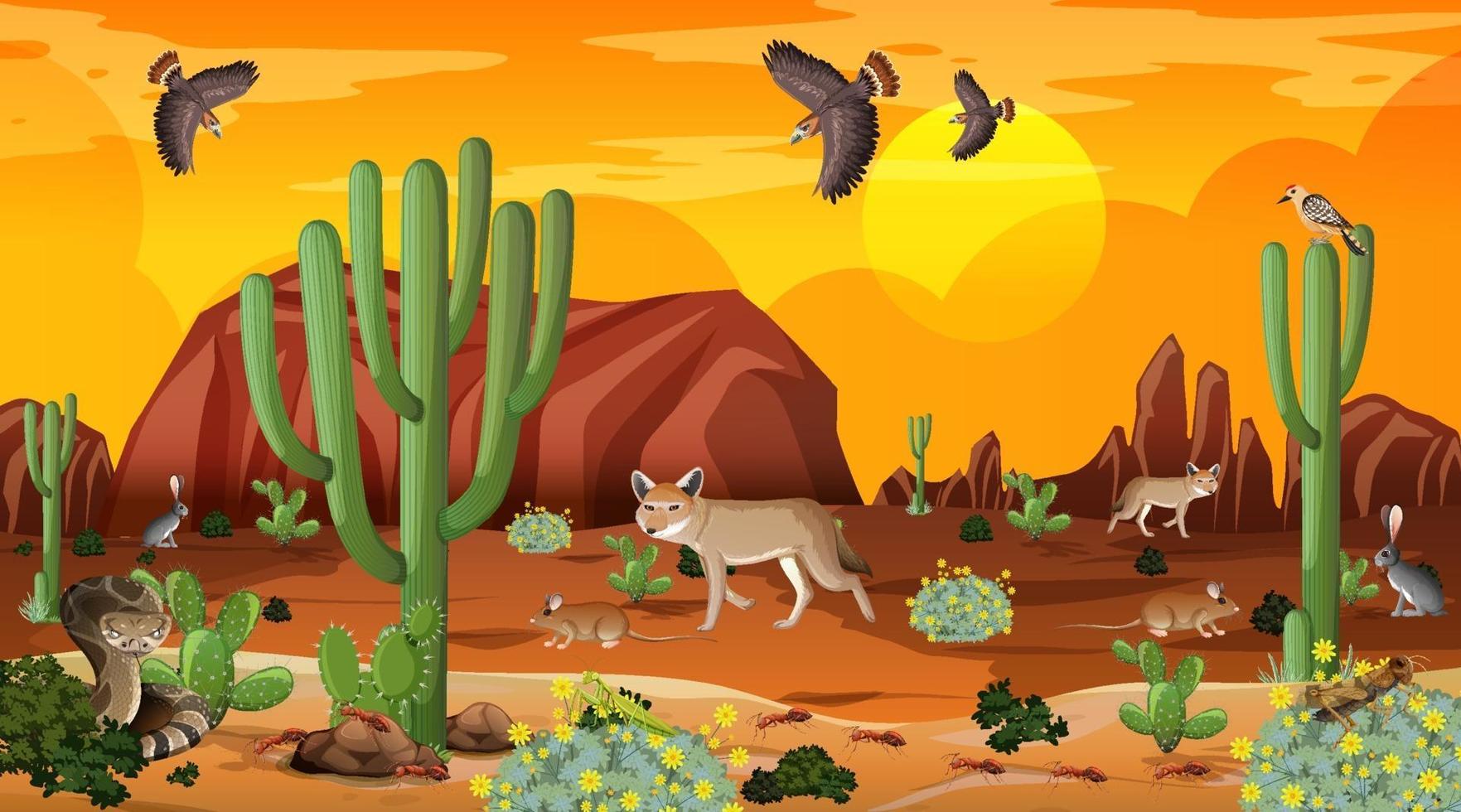This cartoon-style, semi-flat, possibly computer-generated image depicts a desert scene set against a vivid orange and yellow sky, suggesting a sunset. In the center-right of the sky is a golden yellow sun, surrounded by lighter yellow clouds. Three vultures or eagles with brown bodies and red-tail feathers are circling above. The desert landscape is dotted with stereotypical bright green cacti, featuring long, connected segments and smaller circular cacti with visible spikes beneath them. There are bushes and yellow-flowered weeds scattered throughout the scene. On the left side, a large gray and brown cobra is visible, while a rattlesnake is shown further down. The foreground includes a variety of animals: a desert fox near the middle, a fox in the distance on the far right, desert rats, a mouse, and a couple of rabbits. A cricket perches on short vegetation, and fire ants are seen climbing over a rock near one of the cacti. Additionally, a bird rests atop a cactus. In the background are brown rocky plateaus, further emphasizing the arid desert environment.